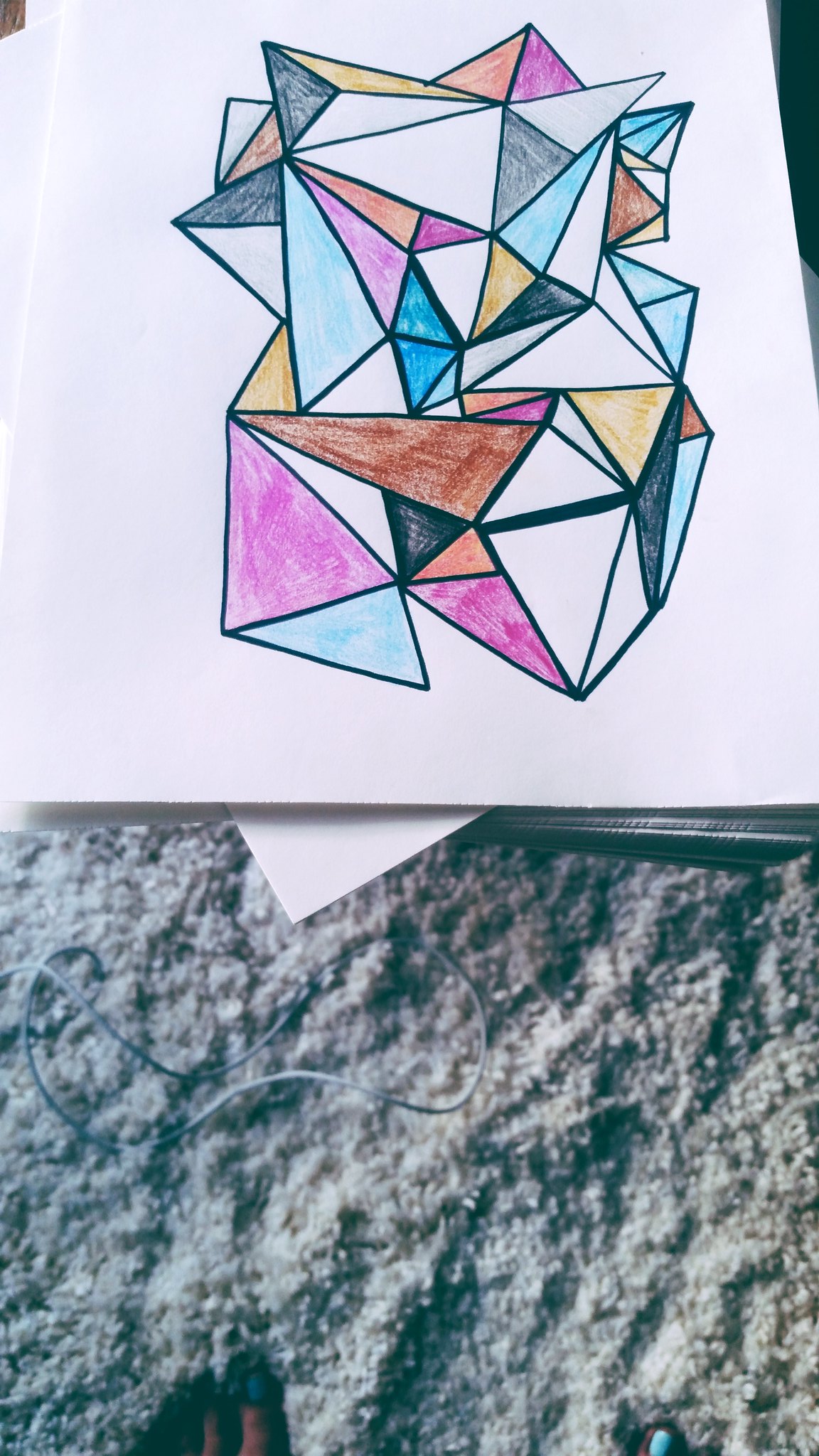The photograph captures a drawing positioned on a table, with the bottom half of the image revealing carpeted flooring and the blue-painted toes of the photographer. The drawing itself is rendered on a white sheet of paper and features an abstract geometric design composed of interconnecting prism-like shapes. The shapes are selectively colored using markers, with hues of pink, blue, brown, and yellow, while some sections remain uncolored. The markers have created an uneven texture in the colored areas, adding an additional layer of visual interest to the composition.